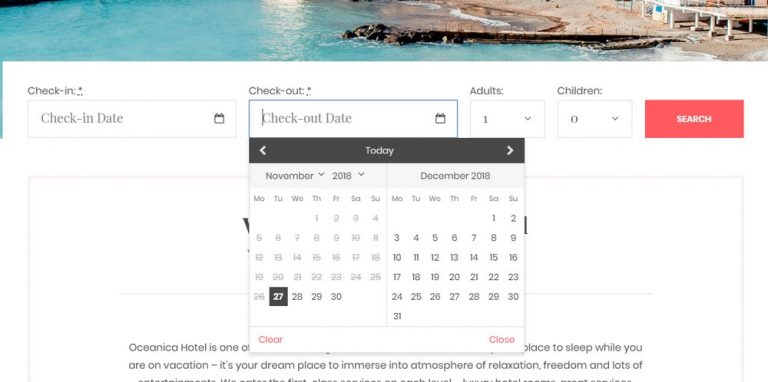The image showcases a section of a website viewed on a screen. The top background features an outdoor photograph taken near the ocean. Visible in the image is a pier extending towards the water, flanked by rocks and sand. A platform or building is situated on the sand near the water's edge. 

Below the photograph, on a white background, the website provides options for check-in date, check-out date, number of adults, number of children, and a prominent red "Search" button with white text. Most of the text on the page is in black font. The user has selected the check-out date option, revealing a calendar interface. This calendar has a black banner at the top that indicates the current day, supplemented by navigation arrows on either side to switch between months. 

The calendar is divided into two sections: November 2018 on the left and December 2018 on the right. The user has selected November 27th, which is highlighted with a black box, differentiating it from the other dates. Red buttons labeled "Clear" and "Close" are located at the bottom of the calendar interface. Behind the pop-up calendar, there is partial text about the hotel, which is identified as the Oceanica Hotel, along with a brief description introducing the establishment.